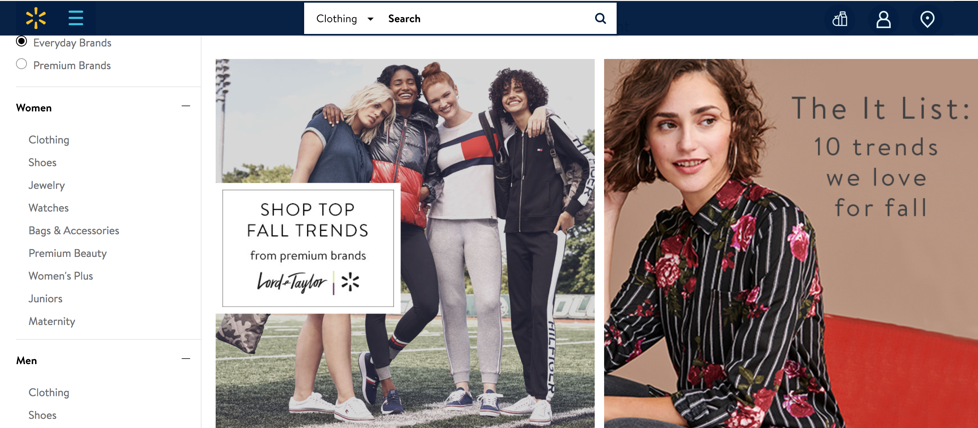The image depicts a webpage from the Walmart website, as indicated by the recognizable Walmart logo in the upper left-hand corner. The top section features a blue banner with several key elements. On the far left, there is the Walmart yellow logo, followed by three parallel lines representing the menu options. Centrally positioned within the blue bar is a search field set to the clothing department. On the far right of the banner, there are icons for location services, account access, and an unidentified third icon.

Below the banner, the main content area consists of two prominent tiles, each featuring a photograph. The left tile showcases a group of four girls posing together in various outfits, accompanied by a tag that reads, "Shop Top Fall Trends by Lord & Taylor." The right tile displays an image of a woman wearing a black blouse adorned with gray stripes and floral designs, labeled "The It List: 10 Trends We Love for Fall."

The left sidebar provides filtering options, with the "Everyday Brands" radio button currently selected. This section allows navigation through categories such as women's clothing, shoes, jewelry, watches, bags, accessories, and more. Below the women's section, there is a similar dropdown for men's categories.